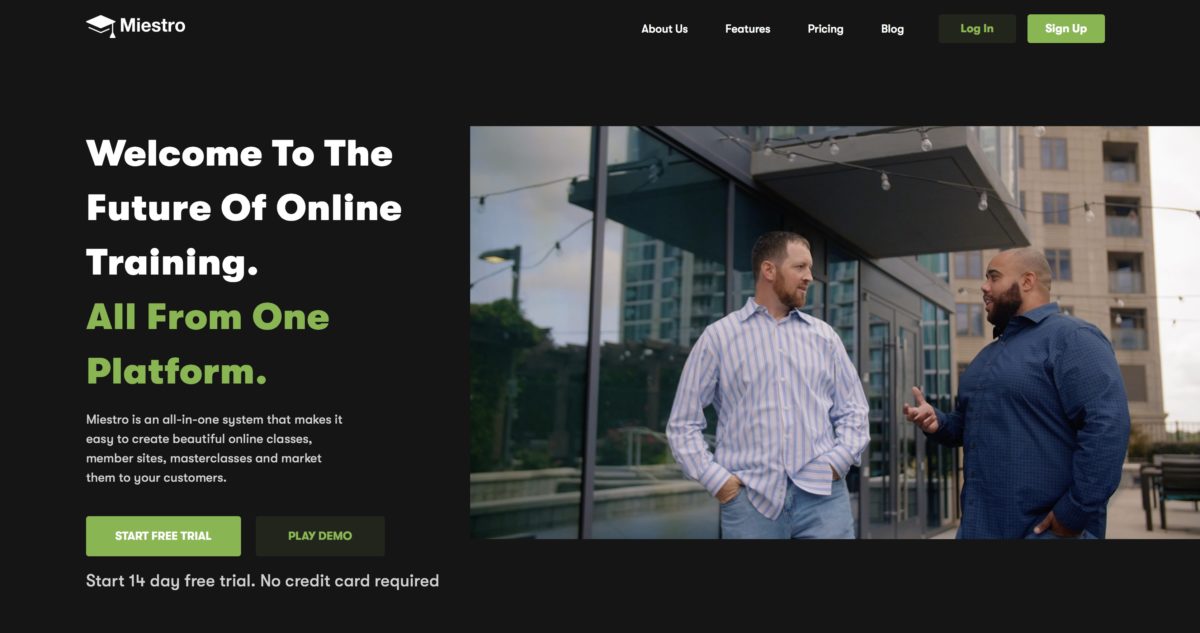The image showcases a screenshot from a website with a sleek black background. In the upper left corner, the website's name "Maestro" is prominently displayed in white text, accompanied by their logo - a white graduate cap. The top right section features a navigation menu with buttons arranged as follows: "About Us," "Features," "Pricing," "Log," a black button with green text for "Login," and a green button with white text labeled "Sign Up."

Below this menu, on the right side, there is a photograph featuring two men engaged in a conversation outdoors. They are standing in front of a tall apartment building during daytime. The man on the left is Caucasian, with brown hair, a beard, and a mustache. He is dressed in a white pinstripe long-sleeved collared shirt and jeans. The man on the right has brown skin, a beard, and a shaved head. He is wearing a blue long-sleeved collared shirt.

To the left of the photograph, in bold white text, the slogan "Welcome to the Future of Online Training" is prominently displayed.